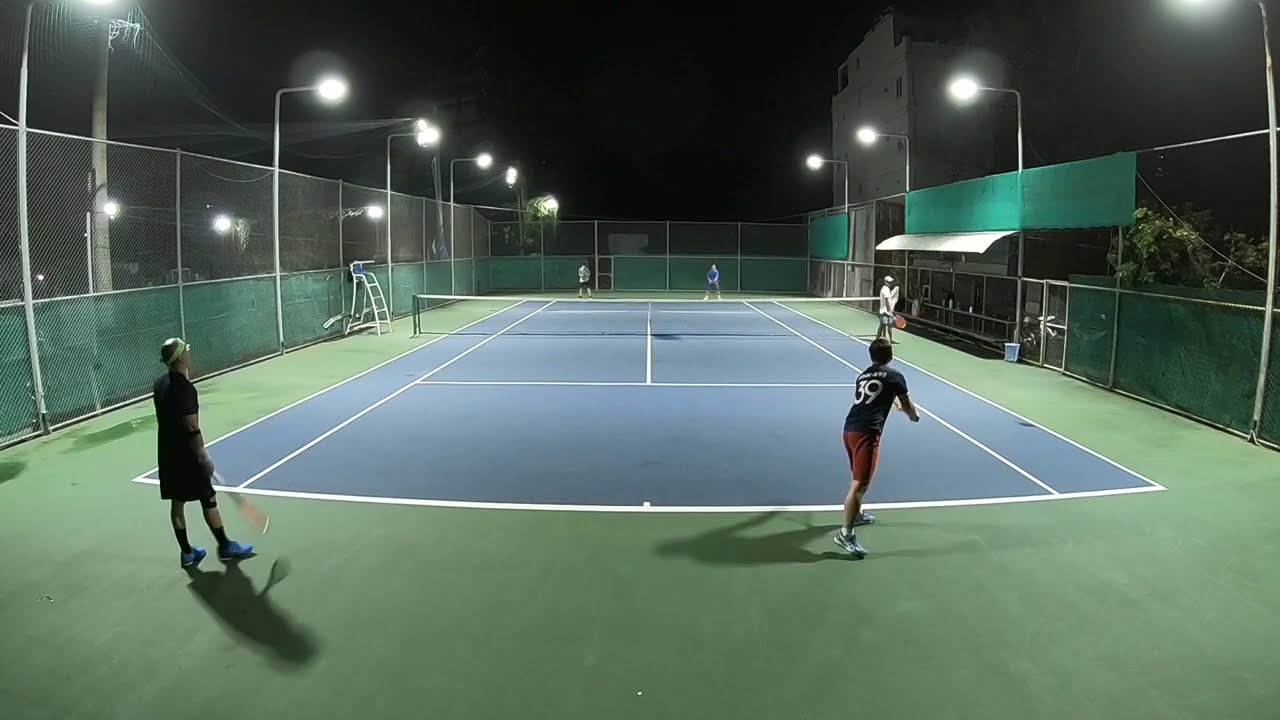The image depicts an outdoor tennis court at night, bathed in the bright illumination of multiple stadium lights positioned around the perimeter. The court surface is distinctively painted bluish with crisp white lines marking the playing areas and enclosed by a green fence. On the court, a doubles match is underway with all four players positioned at the baselines. Closest to the viewer, one player, wearing red shorts and the number 39 on his back, is in a serving stance, slightly bent forward with his right arm extending and his body twisted left. His partner stands nearby, casually holding his racket. On the far side, their opponents are similarly at the baseline, poised to receive the serve. The scene also features some structures: a tall building just right of center in the background and a spectator area with seats on the right side of the court, though it's currently empty. A person in white, possibly another player or a ball retriever, stands off to the right of the net. The court surroundings include green netting and an overhang, reinforcing the sense of an enclosed space focused on this nighttime sporting event. Despite some parts of the photo being slightly blurry, indicating motion, the overall scene captures the intensity and setup of an ongoing tennis match under the night sky.